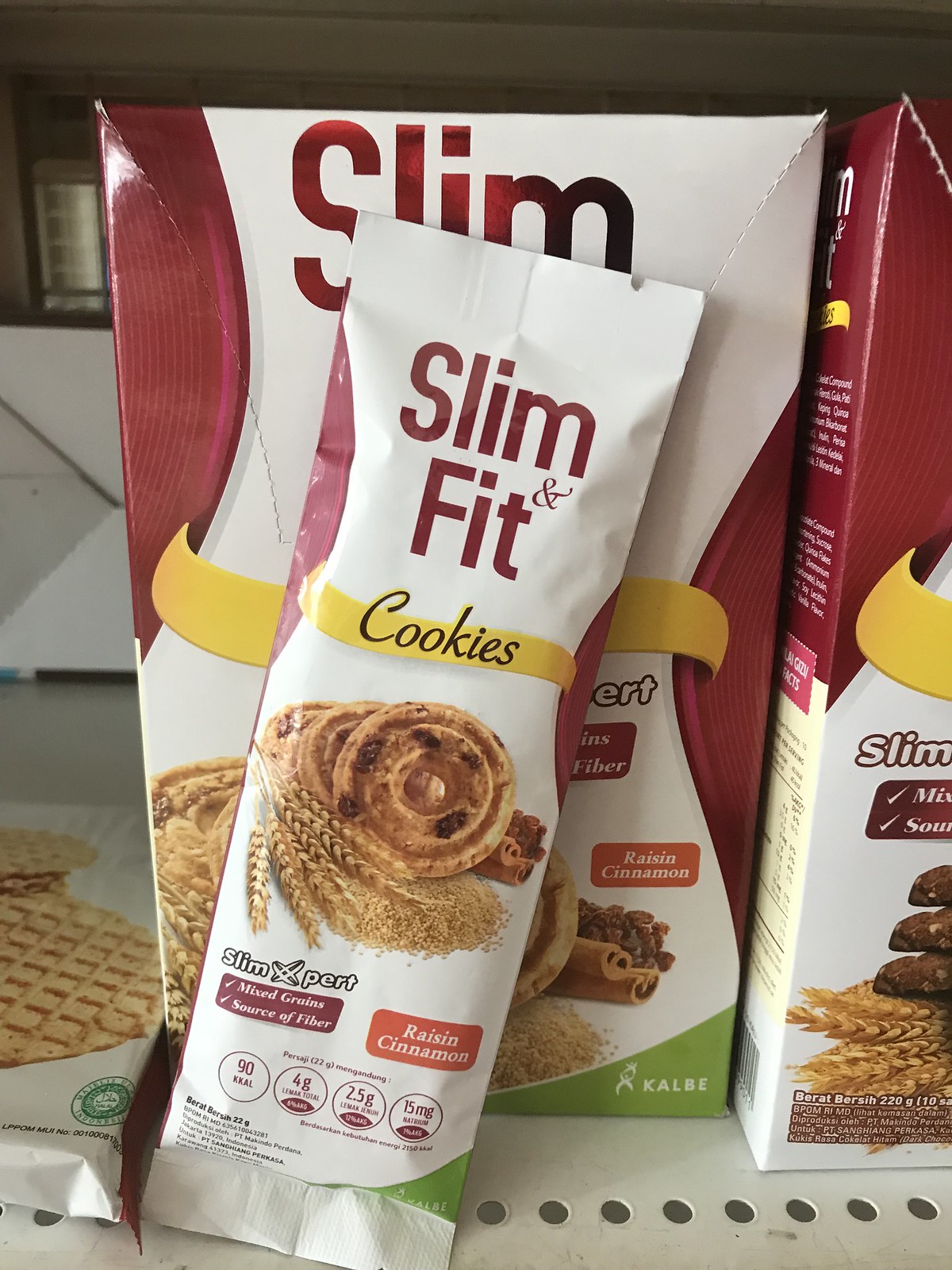The image depicts a retail display of Slim Fit cookies, prominently featuring a single serving pouch and several boxes of the same product in a grocery store setting. The packaging is predominantly white with red text, highlighted by a yellow banner with the word "cookies" written in black. A picture of the cookies along with images of wheat, cinnamon, and raisins is also visible, indicating the raisin cinnamon flavor.

The pouch, standing upright in the foreground, bears detailed yet small nutritional information, noting the cookies as a mixed grain source of fiber, containing 90 calories. The exact values of some nutritional components are hard to discern but include measurements in grams and milligrams. Below this pouch on the shelf, two boxes of the same cookies can be seen, one facing the camera and the other positioned sideways. 

The shelving unit is metal with small circular holes running horizontally, typical of commercial grocery store fixtures. The background shows a portion of a gray floor and a white appliance, suggesting a kitchen display area but primarily focusing on the product itself.

Overall, the display highlights the Slim Fit branding, emphasizing its health-oriented features and the various packaging options available to consumers.